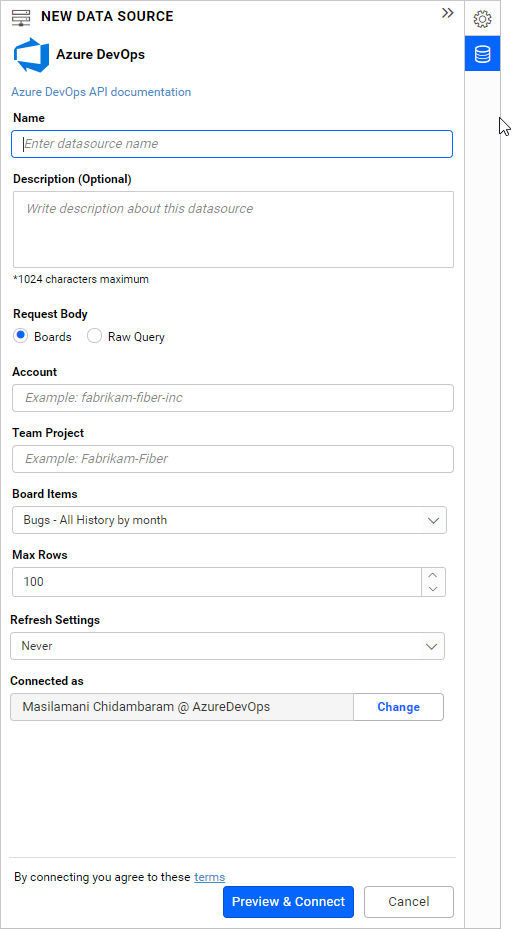The image appears to be a screenshot from a computer interface, specifically from a data source configuration page related to Azure DevOps. In the upper left corner, the heading reads "New Data Source." Beneath this, a white rectangle with a blue border contains the title "Azure DevOps." Following that is a subheading that states "Azure DevOps API Documentation."

The form begins with a field labeled "Name," accompanied by a text box prompting users to "Enter data source name." Below this, there is a section for "Description" marked as optional, featuring a text area where users are invited to "Write description about this data source," with a character limit of 1,024 characters.

Further down, the form includes a subheading "Request Body" with two selectable options underneath: "Boards" and "Raw Query." The "Boards" option is active, indicated by a blue dot next to it.

Additional fields include "Account," with a sample input displayed as "Example: Fabricom Fiber Incorporated," and "Team Project," with an example input of "Example: Fabricom Fiber." There is also a section titled "Board Items," listing options such as "Bugs," "All History by Month," "Max Rows 100," and "Refresh Settings Never."

The interface shows that the user is connected as "Mazalami, Triterbarm at Azure DevOps," and there is a "Change" option on the right side of the screen.